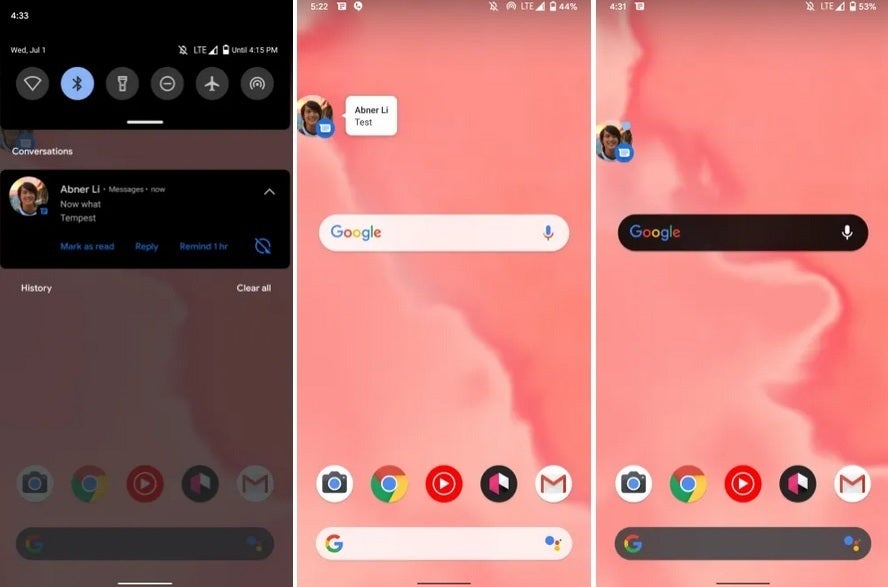This image collage showcases three distinct smartphone home screens, each offering a unique visual theme and layout.

1. **First Home Screen:**
   - **Background:** A solid black color.
   - **Top Section:** Displays the time as "4:33" alongside an instruction that reads "Add one" accompanied by a downward arrow.
   - **Icons & Widgets:** Features a blue box with an insignia, a flashlight, a circle with a dash, an airplane mode icon, and a small target.
   - **Middle Section:** Contains a gray box labeled "Conversations" which includes a profile picture of Abner Lee.
   - **Additional Elements:** Includes a blueprint-like symbol and a circle with a line through it.
   - **Bottom Section:** Shows options for "History" and "Clear All", along with standard icons for functions such as the camera and other utilities.

2. **Second Home Screen:**
   - **Background:** A dreamy pink backdrop with fluffy clouds.
   - **Profile Picture:** Features Abner Lee's picture again.
   - **Icons & Widgets:** Blue box with a shopping cart icon.
   - **Search Functions:** Includes a Google search box.
   - **Bottom Section:** Displays standard smartphone icons and another Google search box.

3. **Third Home Screen:**
   - **Background:** Pink, similar to the second, maintaining a consistent soft aesthetic.
   - **Profile Picture:** Again features Abner Lee's image.
   - **Icons & Widgets:** Repeats the blue circle with a white box resembling a shopping cart icon.
   - **Search Functions:** Displays two Google search boxes in black.
   - **Bottom Section:** Standard icon layout of smartphone functionalities.

This detailed depiction illustrates how the personalized elements and design choices reflect user preferences across different home screen setups.